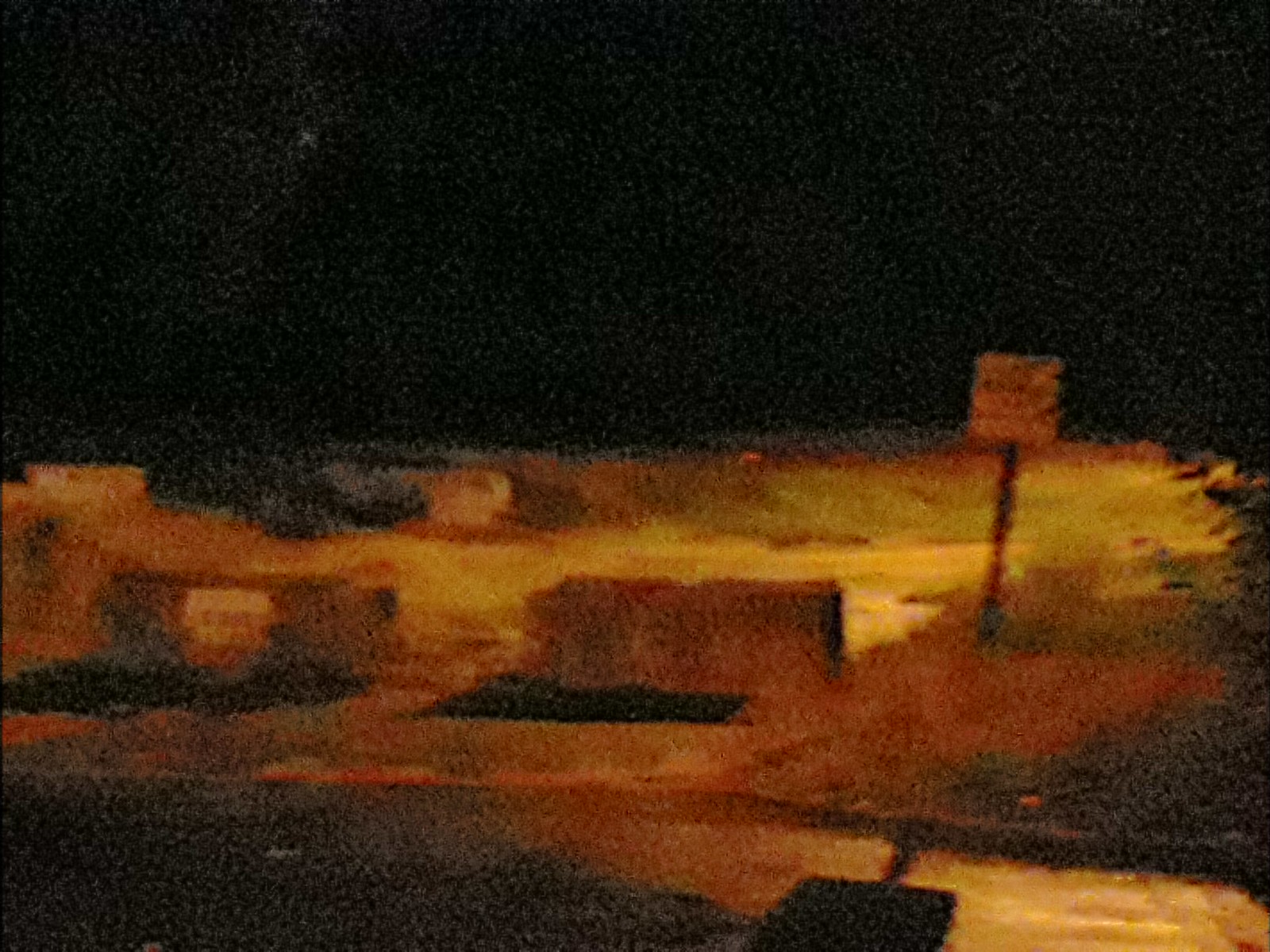The image is a hand-drawn painting, characterized by its very dark and somewhat blurry quality. The upper portion is predominantly black with subtle hints of gray, especially on the left-hand side, where a faint light star dotting the dark sky can be seen. Transitioning to the bottom half, the painting portrays an overgrown parking lot with tall, tan-colored grass. On the far right, there's a bush with additional grass nearby, and the grey outline of a curb is discernible.

Centrally, and slightly left of center, two large, gray concrete dividers are depicted, spaced apart. The left divider has a small white sign, while the right divider features a black post with a white square sign, casting a prominent dark reflection on the black asphalt. The overall setting of the painting exudes an outdoor scene, highlighted by various shades of brown and yellow on the land, and the play of light creating shadows of the signs and dividers on the ground.